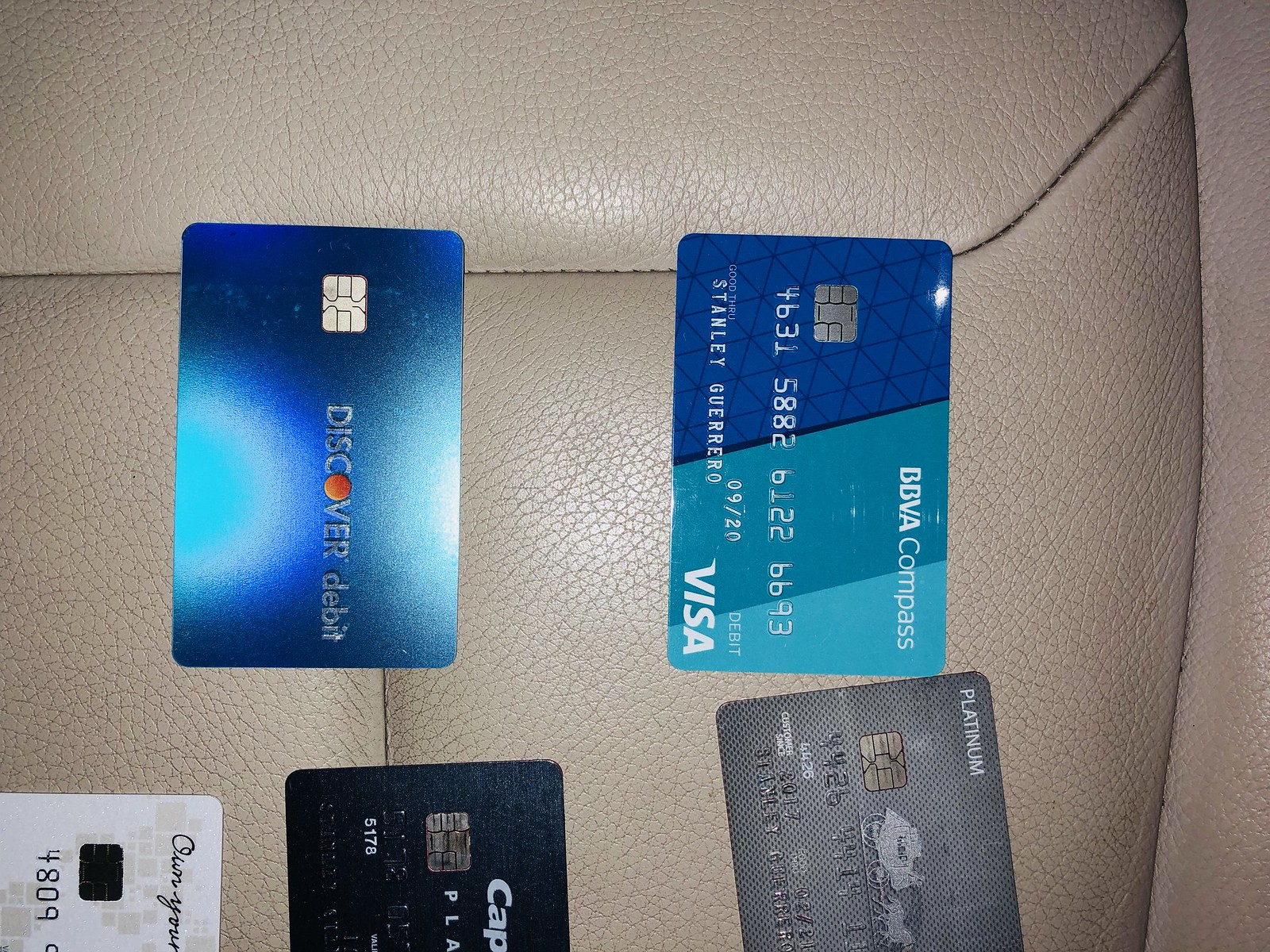The image depicts five credit cards arranged on what appears to be a tan leather car seat, exhibiting stitched sections typical of automotive upholstery. The most prominent cards in the middle include a metallic blue Discover Debit card, featuring a microchip and the distinctive orange "O" in the Discover logo. Adjacent to it lies a BBVA Compass Visa Debit card, characterized by a blue and turquoise gradient, a microchip, and the name Stanley Guerrero, alongside the partially visible card number and expiration date. Below and partially obscured are three other cards: a gray Wells Fargo Platinum card displaying a microchip, a black Capital One card with the visible letters "CAP," and the partially seen white card in the corner, showcasing gray geometric patterns resembling a map of the Americas, and the start of the number 4809.